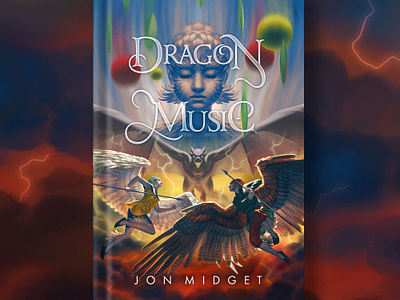In this rectangular image, we are presented with a vividly colorful book set against a striking black and red background. The book, titled "Dragon Music," is prominently displayed in bold white print at the top. The cover artwork is a surreal and fantastical scene that captures the imagination with its rich hues of reds, greens, oranges, and blacks.

At the center of the cover art, there is the head of a young person, their face partially obscured by shadow, adding an air of mystery. Directly beneath this youthful visage is a hybrid creature, appearing to be a fusion of a bat and a human, with its wings dramatically outstretched, commanding attention and lending a sense of dynamic movement.

Below this bat-human figure, two smaller dragon-like creatures with equally pronounced wings are depicted, their forms intricate and mesmerizing. These elements collectively create a layered and fantastical image that draws the viewer in with its complexity and vividness.

Towards the bottom of the cover, the name "John Midget" is clearly printed in white, indicating the author of this intriguing work. The book’s binding is visible on the left side, confirming its orientation. The overall composition of the cover is both enchanting and otherworldly, promising an adventurous and imaginative read.